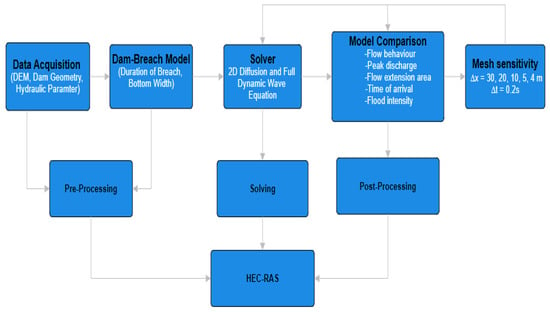This image depicts a meticulously organized flowchart with light blue squares against a white background, interconnected by light gray lines and arrows. The topmost row features five blocks labeled as Data Acquisition, Dam Breach Model, Solver, Model Comparison, and Mesh Sensitivity, from left to right. The second row comprises three blocks labeled Pre-Processing, Solving, and Post-Processing. Arrows indicate connections from Data Acquisition and Dam Breach Model to the Pre-Processing block. The Solver block on the top row points to the Solving block in the second row, while the Model Comparison block connects to the Post-Processing block. At the bottom center, the final block, labeled HEC-RAS, is connected by arrows from all three blocks on the second row, demonstrating a convergence of the processes. The diagram uses a blue, white, and black color scheme, with clear black borders around each square, creating a tidy and easily comprehensible illustration without any additional explanatory text or title.